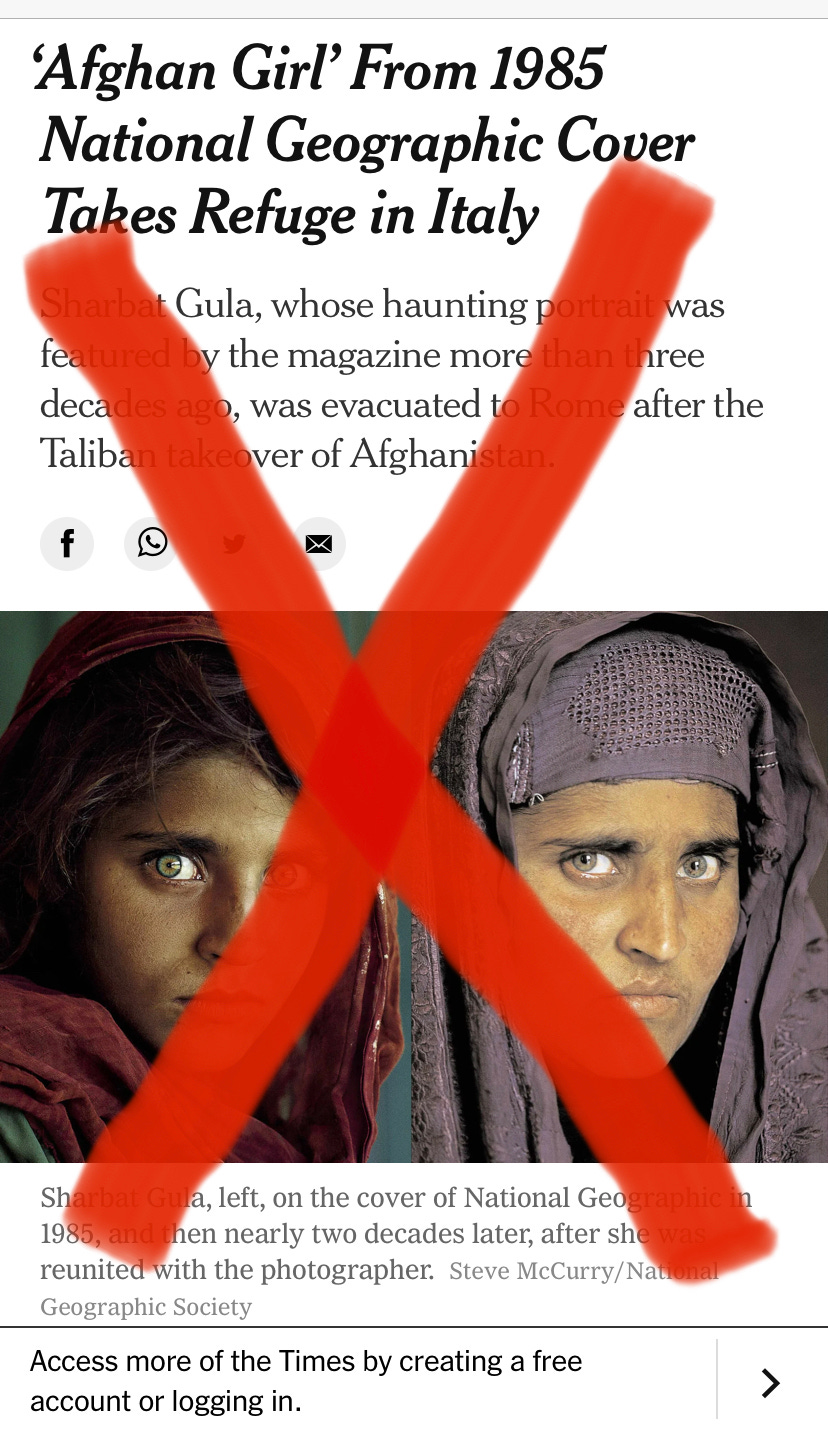The image is a vertically aligned rectangular screenshot from a phone depicting a news article about the renowned Afghan girl from the 1985 National Geographic cover. The article’s headline, written in bold black letters on a white background, reads, "Afghan girl from 1985 National Geographic cover takes refuge in Italy." Below the headline, there are about four lines of text explaining that Sharbat Gula, whose haunting portrait was featured by the magazine over three decades ago, was evacuated to Rome following the Taliban takeover of Afghanistan. 

The main section of the screenshot includes a photograph: it is a side-by-side comparison of the iconic image of Sharbat Gula with her striking green eyes and brown hair on the left, and an older version of her with a gray headdress on the right. A large handwritten red X, as if drawn with a wide-tip marker, covers both the photographs and the accompanying text, suggesting the information might be discredited or false. At the bottom of the screenshot, text encourages users to access more content by creating a free account or logging in, while partially obscured social media icons, including a circular Facebook logo, are visible beneath the red X.